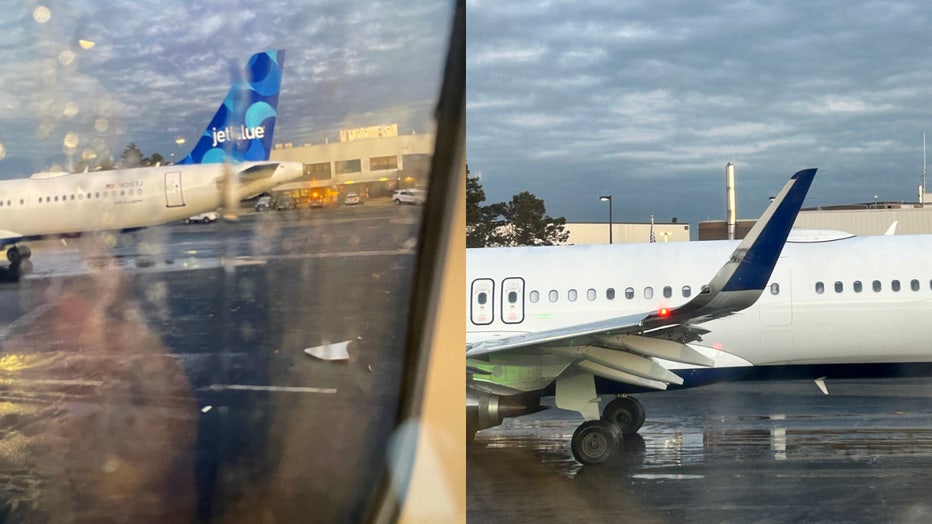The image is a composite of two side-by-side photographs taken from the inside of an airplane. On the left, the photo captures the view through a passenger window, which is speckled with raindrops hinting at recent rain. Outside the window is a JetBlue airplane on the runway, accompanied by several airport carts and a building in the background. The scene is set against a backdrop of gloomy, overcast skies. On the right, the second photo shows a white airplane, likely the same JetBlue aircraft, from a different angle. This view focuses on the middle section of the airplane, displaying its windows, left wing, wheels, and some mechanical components beneath it. The plane is parked on a wet tarmac, with small puddles visible underneath. The cloudy skies persist in this image as well, and a tree is faintly visible to the left side behind the airplane. Both photos jointly create a detailed and atmospheric portrayal of the airplane and its surroundings on a rainy, overcast day.